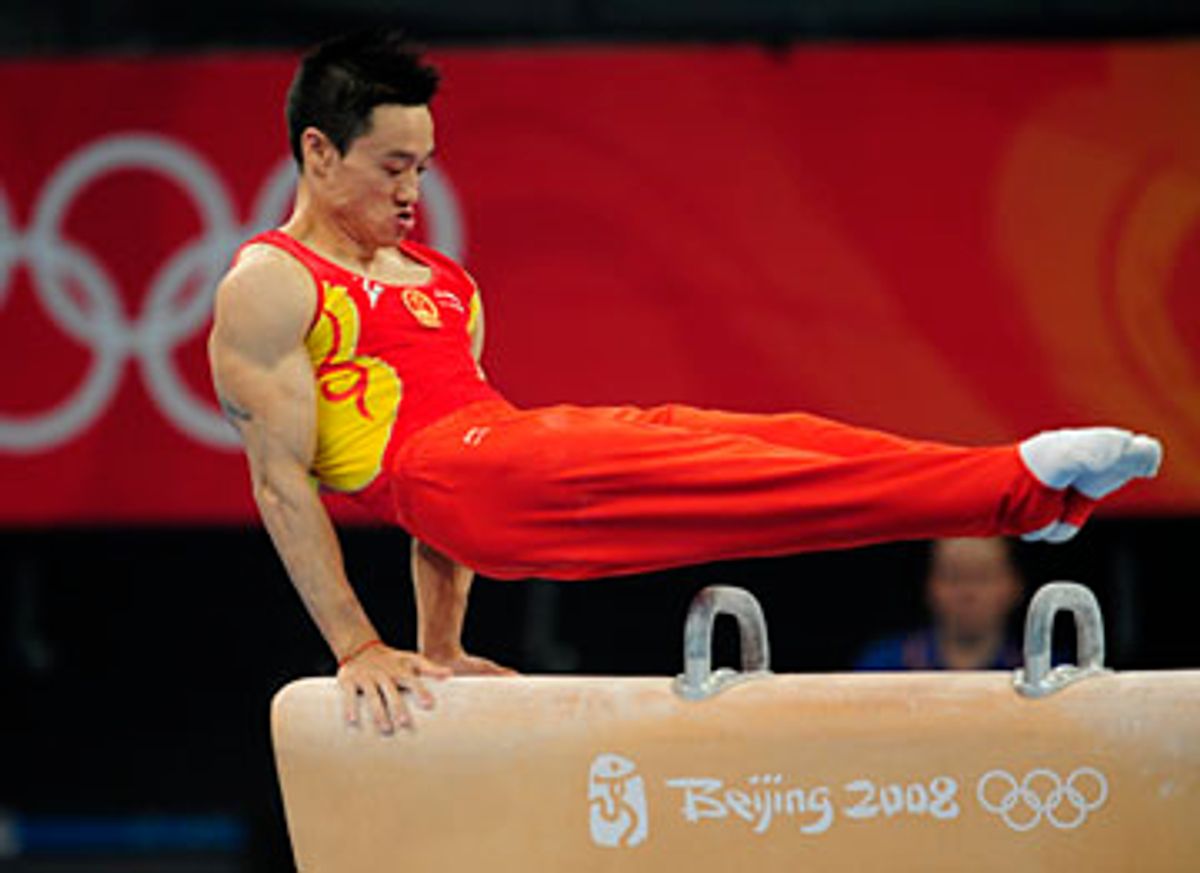This is a horizontal, rectangular photograph capturing a male gymnast from the Chinese team in mid-performance at the Beijing 2008 Olympics. He is performing an impressive move on the pommel horse, not the balance beam as initially thought. The gymnast is sporting a striking red Olympic uniform, consisting of a red tank top with yellow accents and matching red pants featuring white stirrups. He also wears white socks and has short black hair. The athlete displays remarkable strength and control, with his arms muscularly tensed as they support his entire body weight on the beige pommel horse. His hands are firmly grasping the handles of the pommel horse, and his legs are extended straight out horizontally, perfectly rigid and pointed, showcasing his gymnastic prowess. The intense look of concentration and effort on his face highlights the physical demands of his routine. The pommel horse is marked with the words "Beijing 2008" and the Olympic rings in white. In the background, a large red banner featuring the Olympic rings is partially visible, adding a grand and official atmosphere to the image. On the left side of the banner, a distinctive emblem resembling a stylized stick figure is faintly seen, contributing to the overall festive Olympic setting.